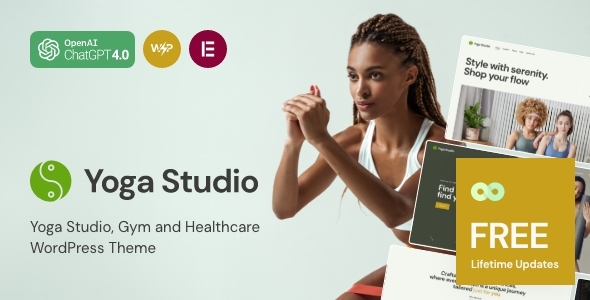The image depicts a promotional banner for a yoga studio that is interspersed with various other related icons and information. The background of the banner is a subtle mint green hue. 

On the top left corner, there is a green banner featuring the white symbol for ChatGPT, accompanied by the text "OpenAI" in white, and just below it, the version number "ChatGPT 4.0."

To the right of this, there is a distinctive yellow icon, leaning towards an orange-yellow shade. The icon displays a white 'W', followed by a lightning bolt, and then a 'P', possibly indicating a WordPress theme. 

Further right, a magenta icon showcases a uniquely separated white 'E', with the left side of the 'E' disconnected from the three horizontal lines on the right. 

Below this, a green icon resembling a yin-yang symbol in white is featured. Directly next to it, in bold dark gray lettering, is the phrase "Yoga Studio." Beneath this, in smaller yet similarly colored text, the words "Yoga Studio, Common Gym, and Healthcare" are written, followed by the phrase "WordPress Theme."

Further to the right, there is a prominent photograph of a woman with dark skin, likely of African descent. She is depicted holding her hands together in a yoga pose, her gaze directed slightly leftward and towards the camera. Her dark hair is intricately braided and styled away from her face. She sports a white V-neck tank top and appears to be positioned on a yoga mat, though the mat is partially obscured by surrounding screenshots.

In the top right corner of the banner, there is a white section featuring an image of two women along with the text "Style, Let's Rendezvous, Shop Your Flow." Beneath this white section, a dark gray background appears with various other text blocks and images. 

To the right edge, an image fragment shows a person who is possibly practicing yoga. Below this, another section contains unreadable text in gray and gold hues.

Centrally positioned above this whole content, a small square icon declares "Free Lifetime Updates" with an adjacent infinity symbol against a greenish-yellow background.